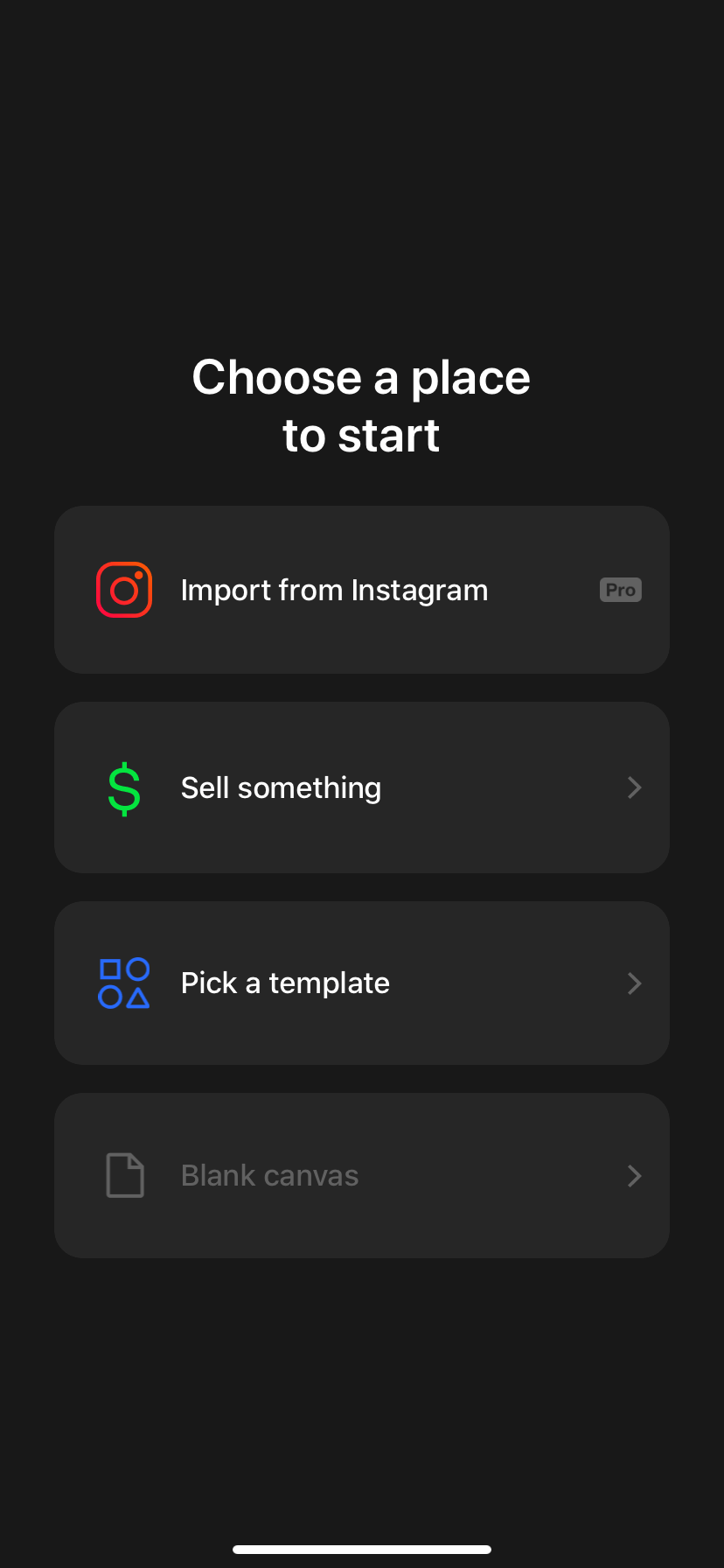This image depicts a vertical, black rectangle that resembles a smartphone screen without any visible device frame. Approximately one-third down from the top, white text reads, "Choose a place to start." Below this prompt are four dark gray rectangular selection boxes, each containing unique icons and text descriptions:

1. The top box features a red Instagram icon on the left, paired with the text "Import from Instagram" in white. Adjacent to this text is a small, light gray box labeled "Pro."
2. The second selection box includes a green dollar sign icon on the left, with the white text "Sell something."
3. The third box displays a unique icon comprising a square, circle, circle, and triangle arranged in a square formation in bright blue. It is accompanied by the text "Pick a template" in white.
4. The final box shows a document icon on the left, with the text "Blank canvas" in light gray.

Each of these gray boxes, except the "Import from Instagram" option, features a forward arrow on the right. At the very bottom of the screen stretches a bold white line across the middle of the bottom edge.